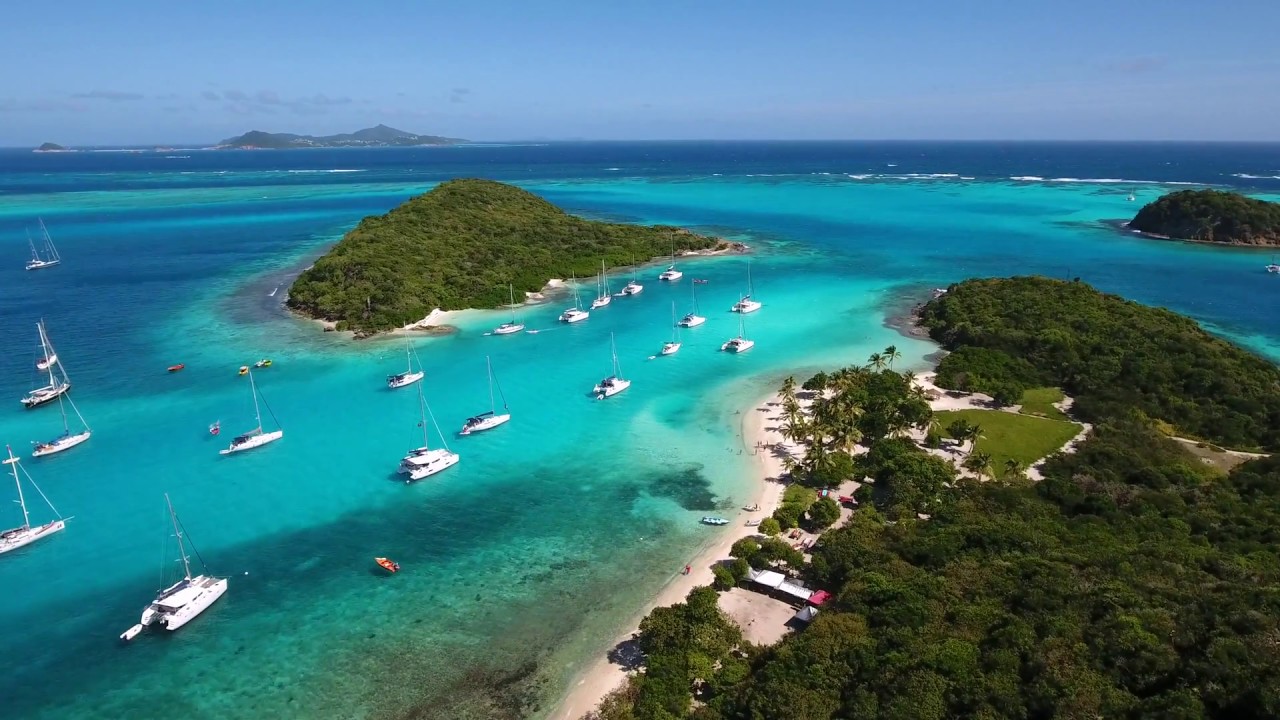This is a stunning aerial photograph showcasing a vibrant tropical island, likely adjacent to a remote resort area. The main island is carpeted with lush green trees and bordered by a thin strip of pristine white sand beach. The coastline is dotted with numerous sailboats and yachts, lined up in neat rows, hinting at a popular mooring spot for visitors. On the island, amidst abundant palm trees, there is a trace of civilization marked by a pink structure, likely part of a house or restaurant, and a red car, alongside a few figures walking along the beach. The crystalline turquoise water reveals the ocean floor beneath, transitioning to patches of darker blue further out. In the background, other green-flora-clad islands rise with gentle hills, casting a serene horizon beneath a clear blue sky.